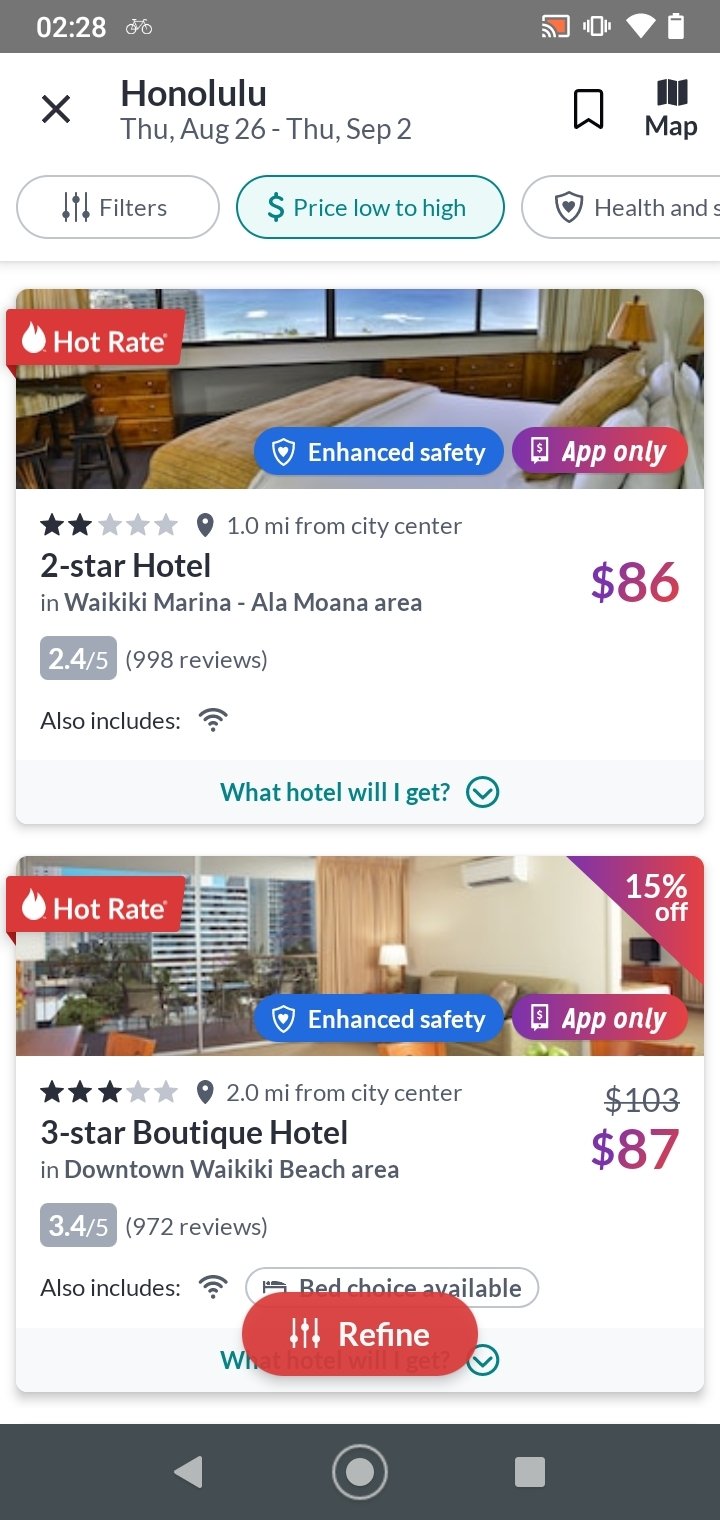The image depicts a mobile phone screen displaying a hotel search interface for a stay in Honolulu. The search details specify dates from Thursday, August 26, to Thursday, September 2. Below the search bar, there are active filters: "Price: Low to High" and a partially visible option related to health standards. 

At the top search result is a listing for a two-star hotel located one mile from the city center, specifically in the Waikiki Marina Ala Moana area. This hotel has a rating of 2.4 out of 5 stars based on 998 reviews and offers amenities including Wi-Fi, as indicated by an icon. The nightly rate for this hotel is $86. 

The next listing is for a three-star boutique hotel priced at $87 per night. The interface provides detailed visuals and relevant information to help users compare and choose accommodations based on their preferences and budget.